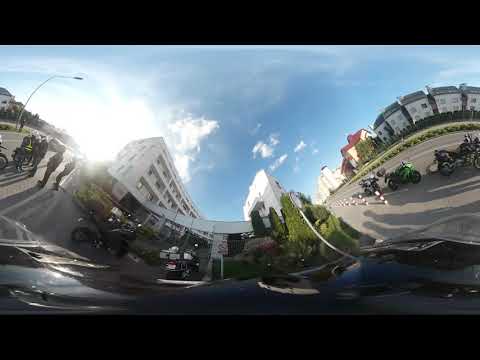This vertical rectangular image features a distorted, fisheye view of a bustling city street, framed by horizontal black stripes at the top and bottom. The street, paved with dark gray concrete, has a dynamic mix of activity and architecture. On the left, a group of people, including a figure who appears to be a police officer wearing a dark green visibility vest, congregates near several parked motorcycles on the sidewalk. A white concrete building with a bordered bridge that extends leftward can be seen behind them, adjacent to a sloping hill.

In the central portion of the image, blurred cars drive along the street, which slopes gently upwards. A commercial building dominates the middle ground, appearing as a single-story structure in the foreground but revealing additional levels in the background. More motorcycles are parked in front of this building, accompanied by some trees that add a touch of greenery to the urban scene.

On the right side, the street is lined with identical tall white concrete buildings, along with a smaller cream-colored building topped with a red roof. A row of either homes or apartments stretches towards the horizon, with numerous parked motorcycles adding to the vibrant urban tableau. The entire scene is set against a backdrop of a blue sky dotted with white clouds, featuring taller buildings just to the right of the center, contributing to the architectural diversity. The image’s curvature and slight blur suggest it might have been captured with a dashcam, giving it a unique, smushed-together appearance.